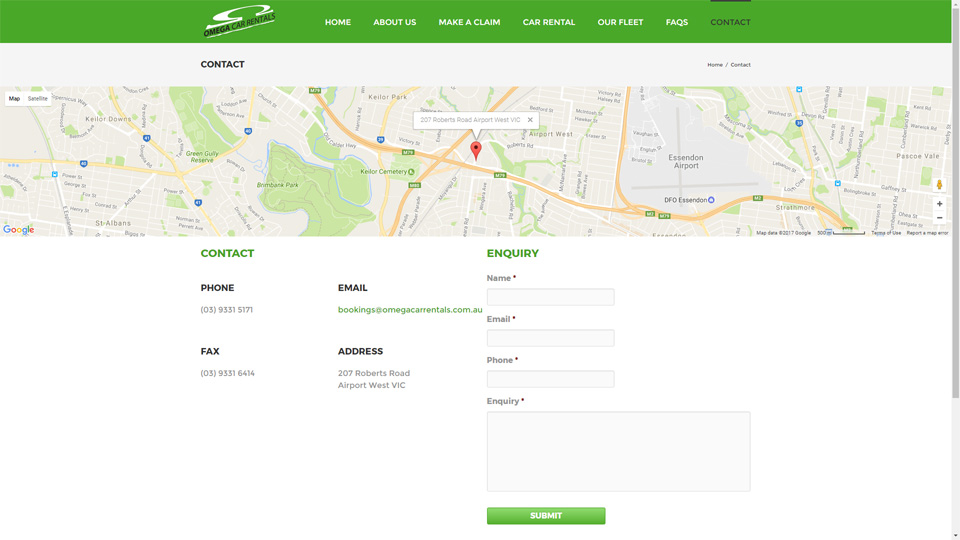Screenshot Description of the Omega Car Rentals Website

This image is a comprehensive screenshot of the Omega Car Rentals website interface. At the top of the page is a toolbar featuring a striking shamrock green color. Positioned on the left side of the toolbar is the Omega Car Rentals logo. The toolbar includes several navigation options listed from left to right: Home, About Us, Make a Claim, Car Rental, Our Fleet, FAQs, and Contact, with the Contact option prominently highlighted.

Below the green toolbar, a white horizontal stripe stretches across the page. The word "Contact" is displayed in black on the left side of this stripe, while both a Home button and a Contact button are situated towards the right.

The center section of the webpage features a large map with a prominent red pin marking a location, presumably indicating the rental office's position. Directly beneath the map, the word "Contact" is rendered in green, accompanied by various contact details. These include a telephone number (not fully visible in the screenshot), an email address listed as Bookings@OmegaCarRentals.com.au, a fax number, and a full physical address: 207 Roberts Road, Airport West, VIC.

Further down the page, there is an Enquiry section complete with text boxes for entering a name, email address, phone number, and the specific enquiry. A green Submit button, matching the toolbar’s color, allows users to send their enquiries directly through the site.

On the right-hand side of the webpage, the page slider is visible and positioned at the very top, indicating that the screenshot captures the uppermost portion of the webpage. Overall, the page is a clean and neatly organized contact section of the Omega Car Rentals website.